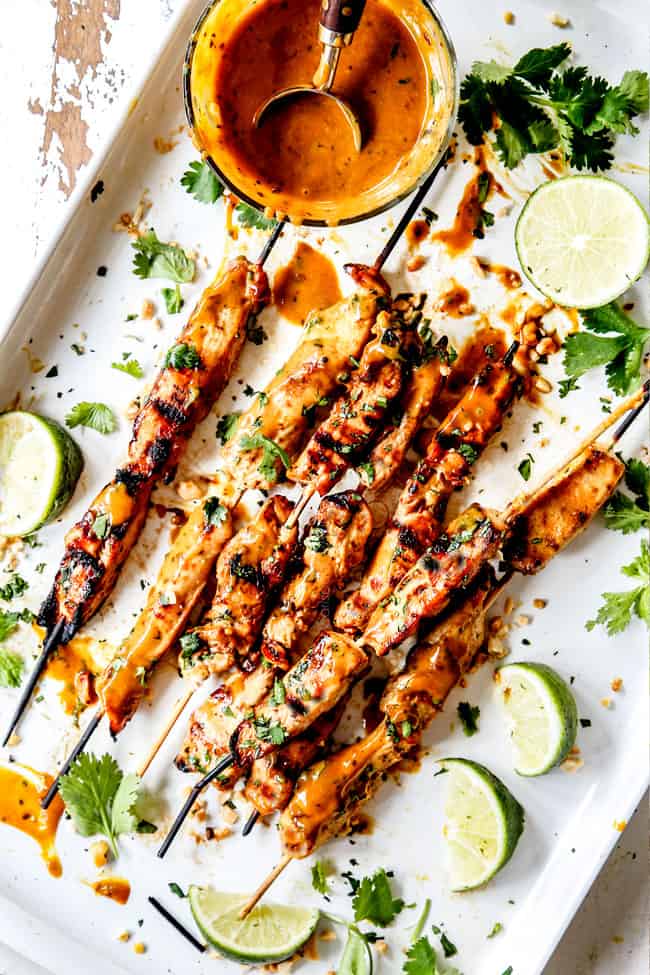This top-down, slightly slanted image showcases a vibrant and appetizing food scene centered on a white metal tray placed on a chipped, wooden table. The focal point is a plate of barbecued chicken or pork skewers, neatly arranged on wooden sticks. The skewers feature a dark golden brown, grilled exterior, and there are six to ten pieces in total. The dish is generously garnished with fresh cilantro leaves and lime slices, some quartered and some halved, adding a bright green contrast to the scene. Accompanying the skewers is a bowl with a rich, orange-colored satay or peanut sauce, speckled with darker bits, creating a visually appealing mix. The overall presentation, though slightly messy, emanates a rustic charm that enhances its mouth-watering allure.